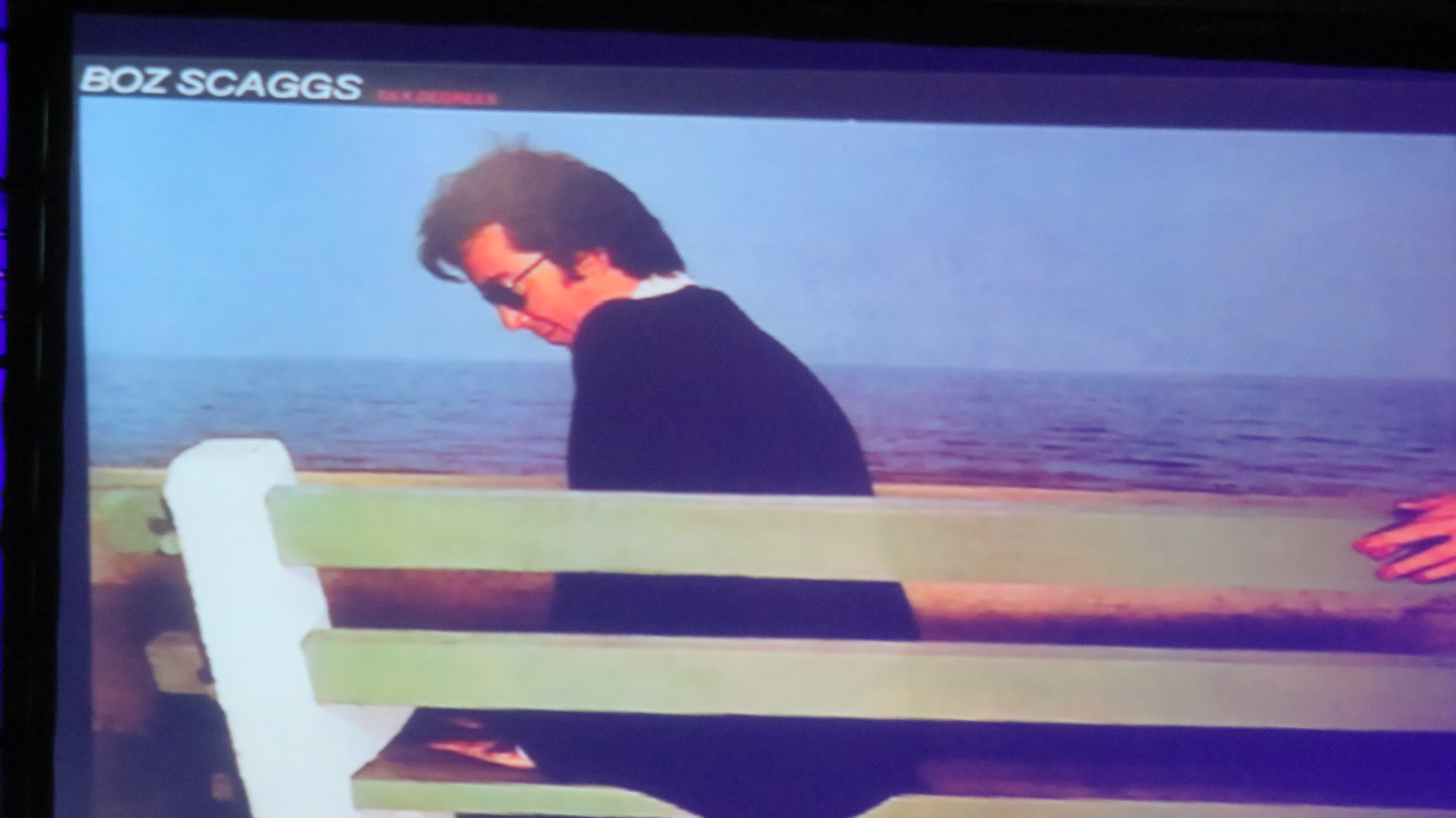The image is a screenshot from a movie, capturing a scene displayed on a screen, possibly a computer monitor or tablet, identifiable by the black bezel and border around the screen. The film features a man sitting on a white-painted bench near an expansive body of water, which appears to be a sea or ocean extending as far as the eye can see. The man, who has short, shaggy brown hair and dark sunglasses, is facing left. He is dressed in a black suit with a bit of a white dressy shirt visible around the neck. Notably, there is a caption at the top left of the screen that reads "Boz Skaggs." The scene also includes a detail of someone's left hand resting on the top of the bench.